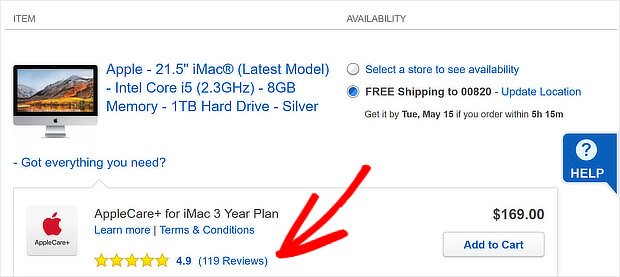The image features a pristine white background with a prominent rectangular box outlined in gray. This box is divided into two sections by a slightly darker horizontal line. In the upper left corner, bold capital letters spell out "ITEM," and directly to the right, it reads "AVAILABILITY." Below this header, an image of a computer monitor is displayed. The monitor shows a beautiful landscape featuring a lake, autumn foliage, and distant mountains as its wallpaper. 

Beneath the monitor image, detailed specifications for the device are listed: "Apple 21.5 iMac, latest model, Intel Core i5 2.3 GHz, 8 GB memory, 1 TB hard drive, silver." Under this description, another box is present, displaying the AppleCare logo on the left. Adjacent to the logo, text states: "AppleCare Plus for iMac 3-year plan, $169." A hyperlink labeled "Learn More, Terms and Conditions" is provided, along with a rating indicator showing "4.9 stars" based on "119 reviews." A red arrow has been editorially placed, pointing toward the "119 reviews" text, emphasizing this detail.